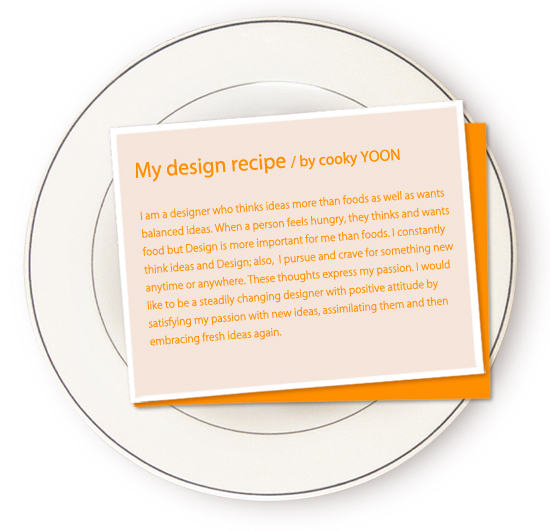The image appears to be an advertisement showcasing a designer's philosophy, presented creatively on a plate. The plate, white with black accents, features two concentric stripes and serves as the background for two layered cards. The bottom card is a rich yellowish-orange, partially visible to the right and underneath the top card. The top card has a pinkish white background with vibrant orange text that reads: "My Design Recipe by Cookie Yoon." Below, Yoon's message states, "I am a designer who thinks ideas more than foods as well as wants balanced ideas. When a person feels hungry, they think and want food, but design is more important to me than foods. I constantly think ideas and design. Also, I pursue and crave something new anytime or anywhere. These thoughts express my passion. I would like to be a steadily changing designer with a positive attitude by satisfying my passion with new ideas, assimilating them, and then embracing fresh ideas again." The text uniformly emphasizes Yoon's dedication to design and innovation, neatly framed within the aesthetic presentation.